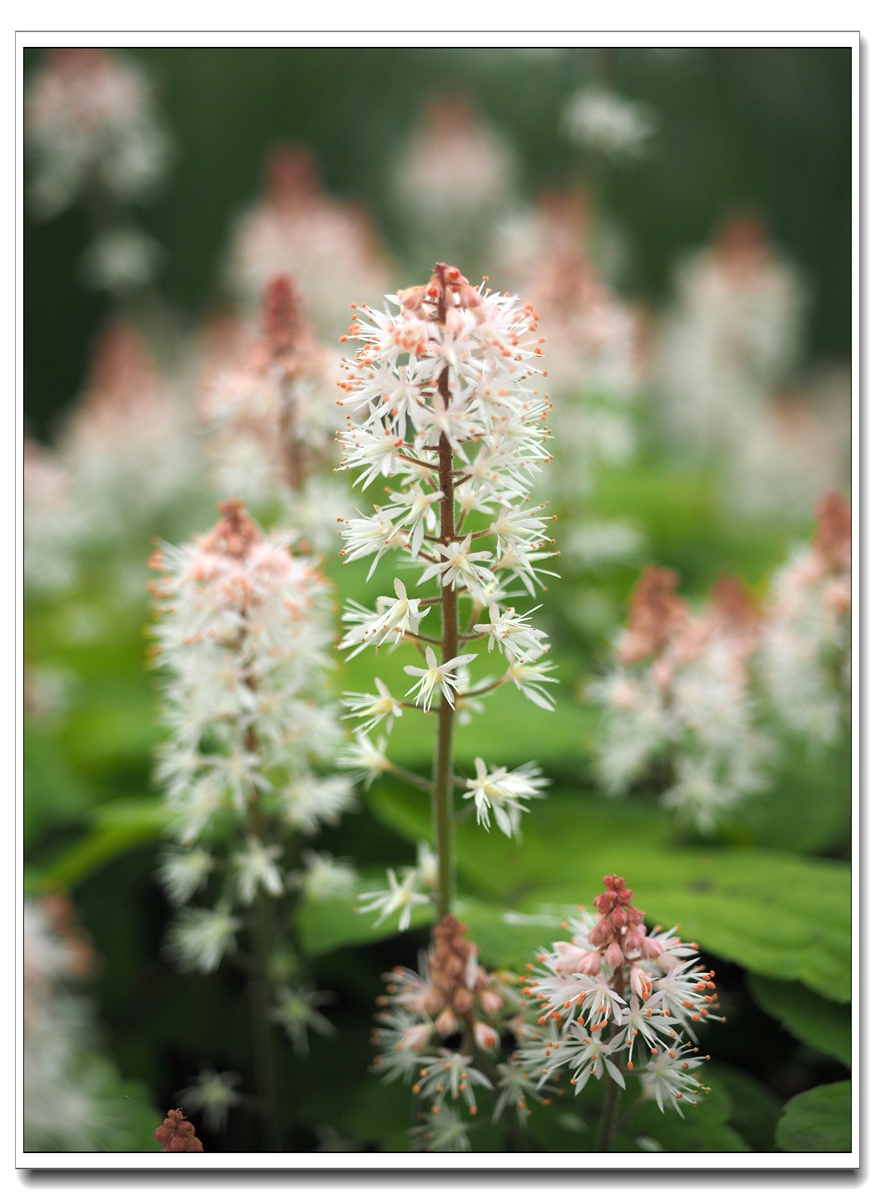The image captures a striking white flower with an elongated stem, adorned with numerous delicate white blossoms. Each flower is intricately detailed, with the petals giving way to subtle purple or brownish hues at their tips, adding a fascinating contrast to the overall pristine white. In the background, a softly blurred scene reveals more of these ethereal flowers, set against a lush green backdrop that enhances their purity and grace. In the foreground, several blossoms are still in the bud stage, characterized by small, round brown buds that promise future blooms. The overall composition exudes natural beauty and the promise of blossoming life.